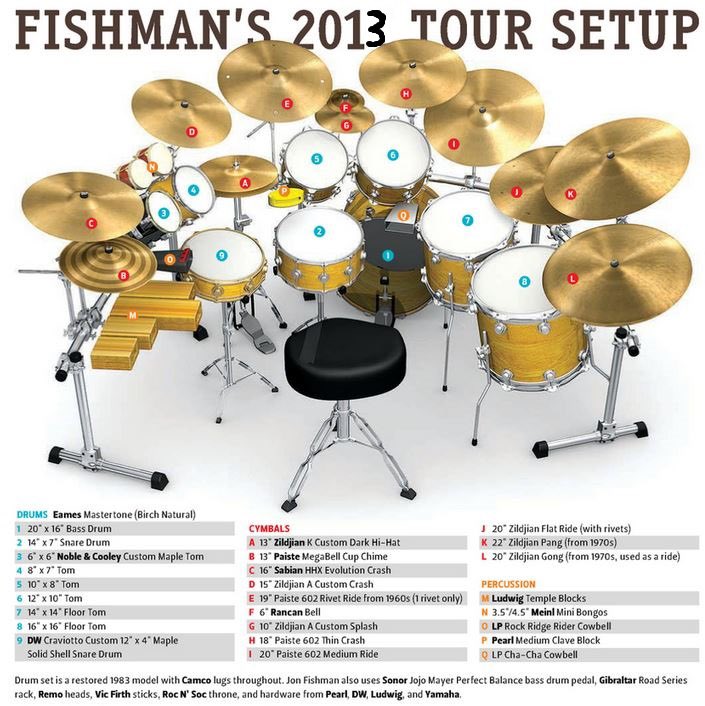This image is a detailed illustration of Fishman's 2023 tour drum setup. At the top in large, bold letters, it reads "Fishman's 2023 Tour Setup." The arrangement features a restored 1983 drum set, meticulously labeled for easy identification. The setup includes around 20 different drums, cymbals, and percussion instruments, each marked with small circles containing numbers or letters—numerical indices in blue and alphabetical indices in red. A black stool for the drummer is centrally positioned. Below the main image, there is an extensive breakdown explaining the category and placement of each labeled drum, cymbal, and percussion piece. Notably, the set incorporates components such as Camco Higs, Sonar drums, a Mojo Mayor Perfect Balance Bass Drum Pedal, a Gibraltar Road Series Rack, Remo Heads, Vic Firth Sticks, a Rockin' Sock Throne, and various hardware from Pearl, DW, Ludwig, and Yamaha.